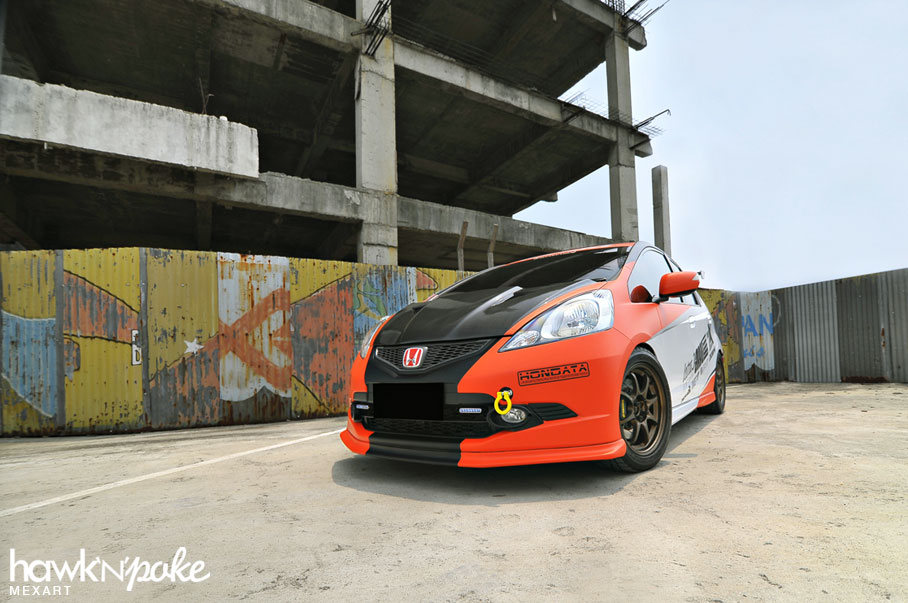This color photograph captures a detailed scene of a small sports car, prominently featuring a Honda Civic. The car, which is predominantly red with a black hood and white side panels accented by black trim and red side mirrors, is parked in a gravel or dirt lot. The front bumper displays the word "Hondata." In the bottom left corner of the image, white text reads "Hawk and Poe Maxart." Behind the car stands a metal fence with patches of paint and sections of plain metal, which is covered in graffiti. Beyond the fence looms the silhouette of a large, featureless building, likely an empty or potentially abandoned parking garage. Positioned in an urban setting under a blue sky, this image juxtaposes the vibrant car with the stark, utilitarian background.